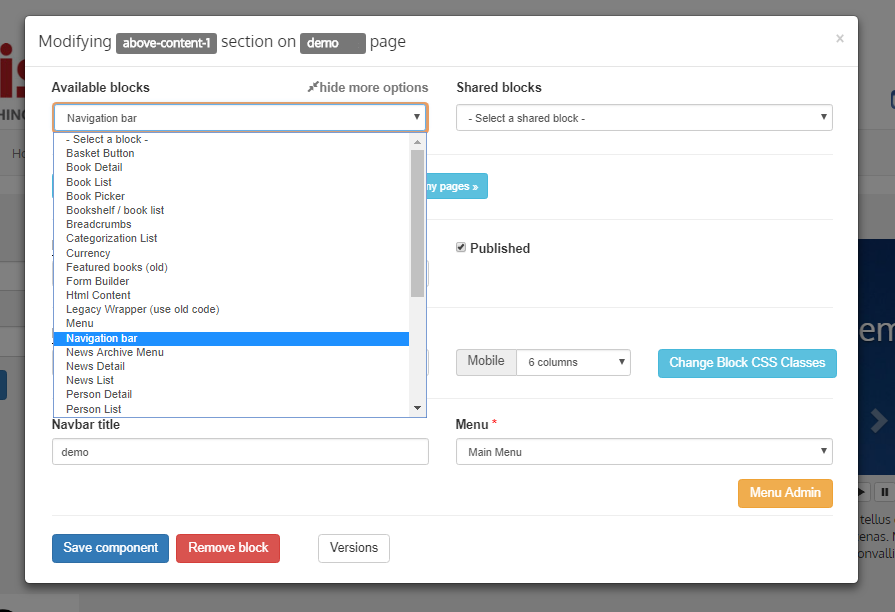The image displays a screenshot of a computer screen featuring a white dialogue box from a webpage customization tool overlaid on the actual webpage. The header at the top of the dialogue box reads "Modifying above content section on demo page." Below the header, there's a gray 'X' for closing the popup. The dialogue box includes a dropdown menu labeled "Available Blocks," which currently has "Navigation Bar" selected and highlighted in blue. This section allows the user to choose from various options such as basket button, book list, categorization list, featured books, form builder, and more.

On the right hand side beneath "Shared Blocks," the options include "Published," which is ticked off, and "Mobile," which is set to "six columns." In the "Menu" section, "Main Menu" is displayed, with a yellow button labeled "Menu Admin" underneath. At the bottom of the box, there is a blue button labeled "Save Component," a red button labeled "Remove Block," and a white button labeled "Versions." This popup interface appears to be a tool for customizing different parts of a website, with functionalities for saving, removing, and managing various blocks and components of the webpage.